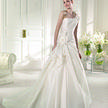This is a small, cropped thumbnail image of a woman in a white, strapless wedding dress that flows down to the floor and pools around her feet. The woman, whose face is partially cut off at the eyes, stands with her arms at her sides in a white room adorned with white carpet and white double doors. To the right side of the image are two white floral bouquets, and to the left, the edge of a white sofa is just visible. The dress appears to have a traditional design, likely made of silk, and is form-fitting around the torso and upper chest. The soft white lighting enhances the serene and elegant atmosphere, suggesting the image might be an advertisement for a bridal magazine or shop.